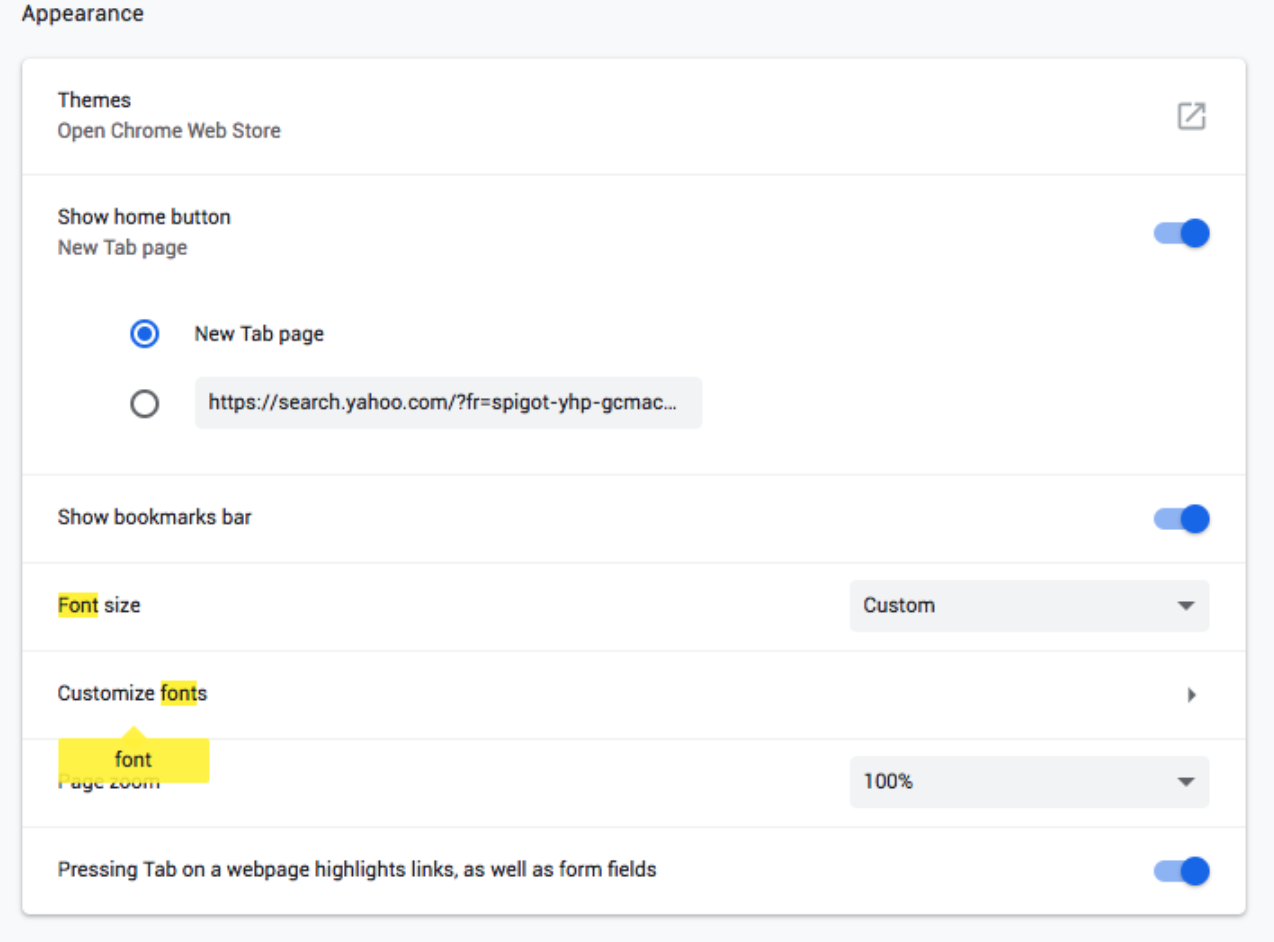The image features a detailed interface of a settings menu, presumably for a browser or operating system. The background of the interface is primarily gray, with nested gray boxes that contain various configurations.

In the top left corner of the primary gray box, there is a section labeled "Appearance." Within this area, you'll find a smaller white box with the word "Themes" displayed in black text, followed by a clickable option titled "Open Chromebook," displayed in gray text. To the far right side of this section, there is an icon of a box with an arrow pointing outward towards the top right, indicating an external link or action.

A dividing line separates this section from the next. Below, black text reads "Show Home Button" next to a toggle button that is switched to the 'on' position. Beneath this, gray text indicates "New Tab Page," accompanied by two selectable options, with "New Tab Page" currently selected. Below this is a text input bar where a URL using Yahoo has been entered.

Further down, another line separates this from the next setting, which reads "Show Bookmarks Bar," toggled on, followed by another separator. Below this, "Font Size" is displayed in black text, with the word "Font" highlighted in yellow. Adjacent to this is a drop-down menu with the option "Custom" selected.

Another dividing line follows, leading to a "Customize Fonts" option where "F-O-N-T" in the word "Fonts" is highlighted in yellow. An adjacent arrow allows for more font customization options.

Below this marked section is another dividing line, and then the label "Page Zoom," leading to yet another separated box, indicating further settings or options.

The overall interface is well-organized, with multiple adjustable settings for appearance and customization, clearly delineated by lines and highlighted indicators for easy navigation.